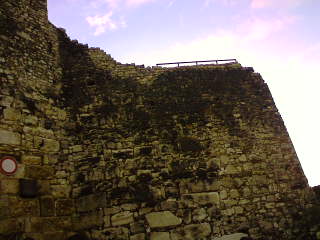In this photograph, we observe a daytime scene of an ancient stone structure that closely resembles a castle wall. The image, possibly no larger than three inches wide and two inches high, captures the view from the base of this formidable stone edifice, looking upwards. The structure's age is evident from the diverse assortment of stones, varying greatly in size and shape, that compose its rugged facade. Some sections of the wall feature large, robust blocks, while others consist of smaller stones intricately stacked together.

A distinctive feature at the top of the wall is a metal railing, seen in the form of five vertical posts connected by a horizontal bar, likely serving as a safety barrier for what appears to be a scenic overlook. At the top and slightly spreading down the wall, patches of moss add a touch of nature to the man-made structure. The wall profile displays a sloping top that descends steeply towards the right before leveling out and then descending sharply again near the bottom right corner.

Backlit by the sun, the wall casts dramatic shadows, with sunlight peeking through and illuminating a bright blue sky adorned with a visually appealing blend of white and pink clouds, transitioning into hues of blue and purple. The scene is void of people, directing all attention to the historical and architectural elements of the stonework and the tranquil, partly cloudy sky that frames the ancient structure.